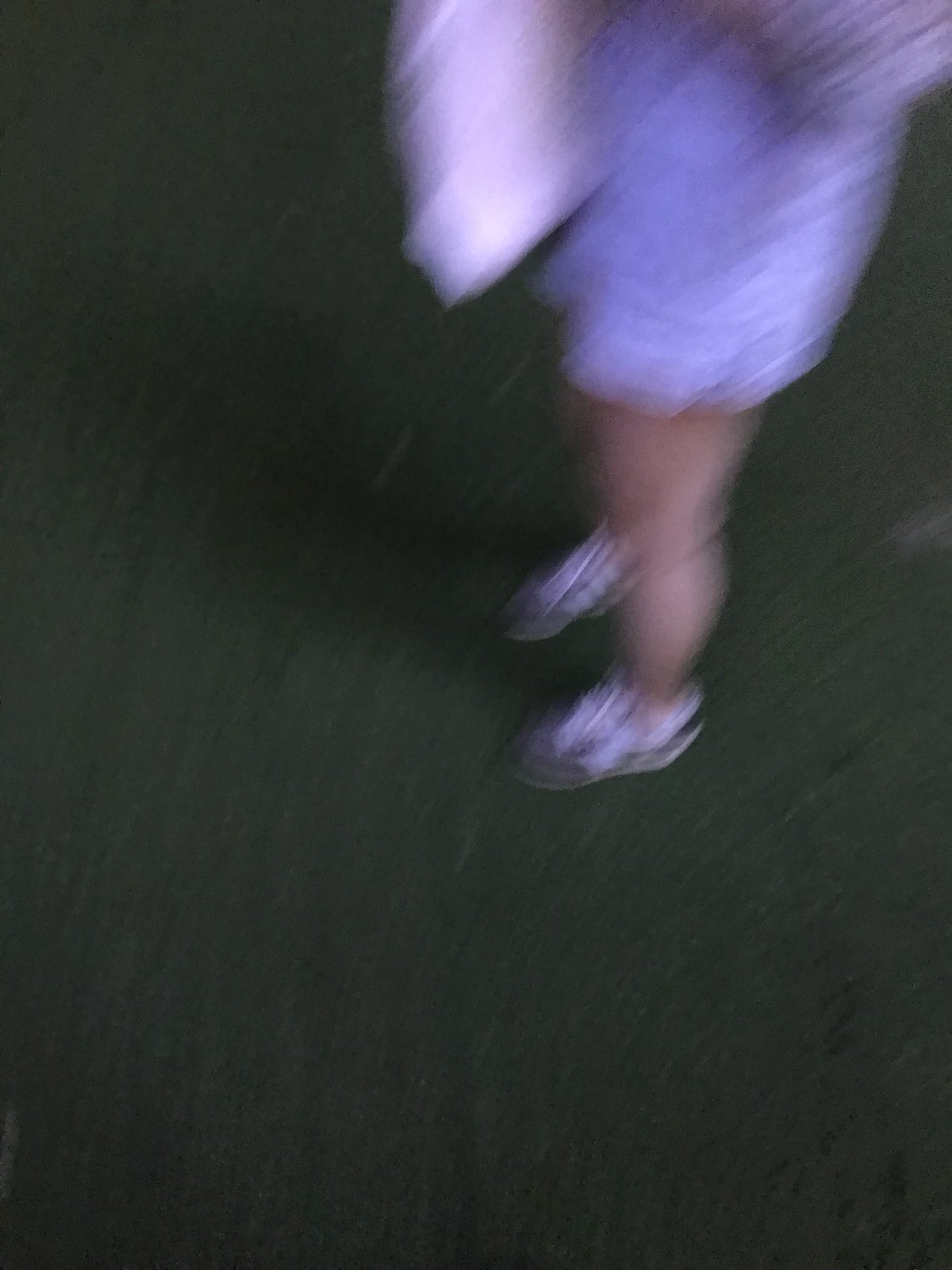A blurred, accidental overhead shot captures a woman's legs standing on a black concrete surface. She is attired in short blue jean shorts and gray shoes, with her light-colored shirt indistinct and blending into the overall soft focus of the image. The woman stands angled with her front facing left, offering a right side view from the waist down. Her left hand clutches a slightly stretched, white bag, while her raised right arm, a blur near her face, suggests movement or an act of shielding or gesturing.